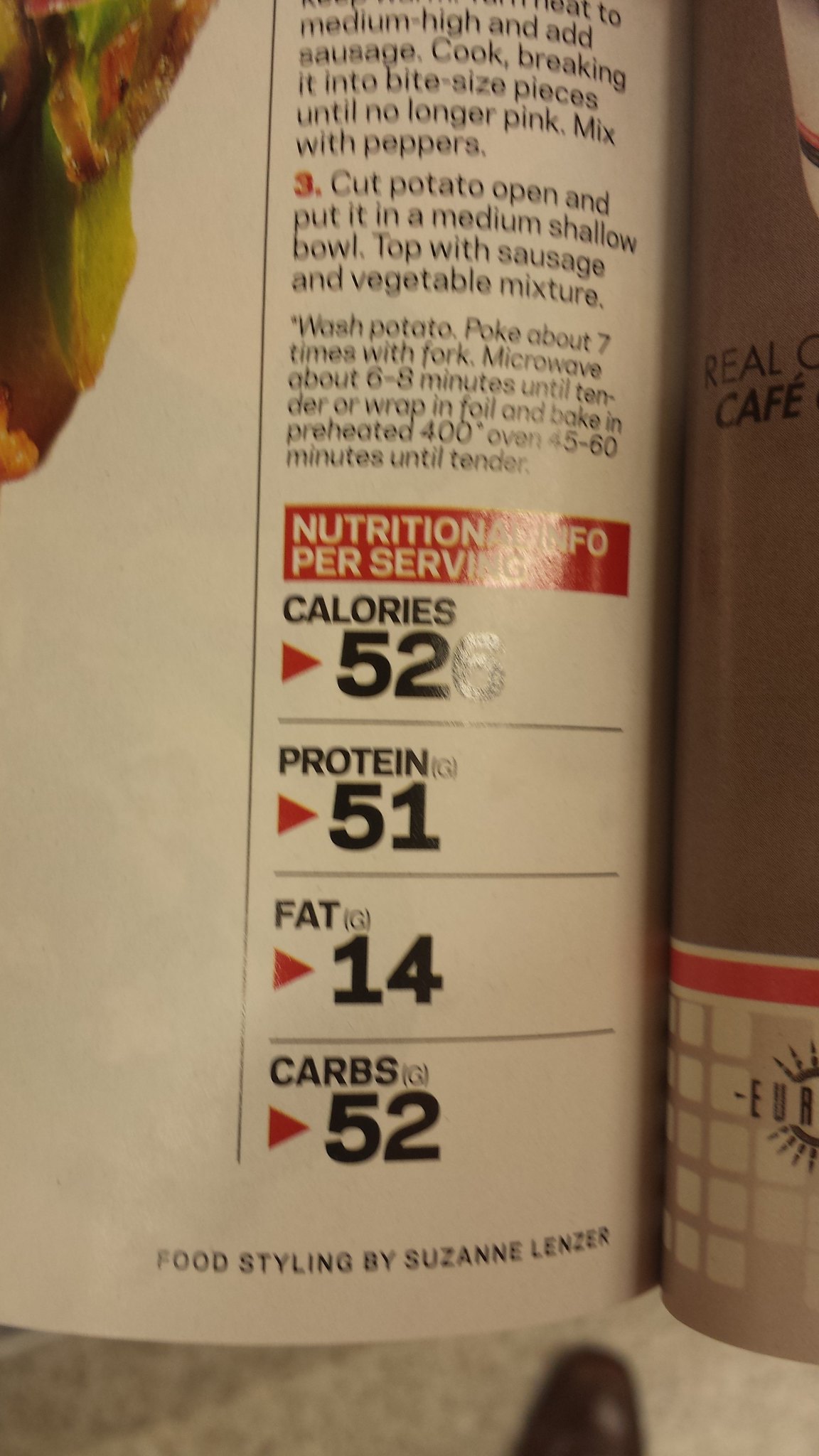This photograph captures a partial recipe page from a magazine titled "Food Styling" by Suzanne Lenzer, as indicated at the bottom of the page. The visible portion includes steps two and three of the recipe, suggesting a detailed and structured cooking process. 

Step two describes cooking sausage over medium-high heat, breaking it into bite-sized pieces, and continuing until it's no longer pink. In step three, the instructions detail cutting open a potato, placing it in a medium shallow bowl, and topping it with the cooked sausage and a vegetable mixture, which was presumably prepared in step one.

Additionally, the nutritional information for the dish is provided: 52 calories, 51 grams of protein, 14 grams of fat, and 52 grams of carbohydrates. The image offers a snapshot of a flavorful and structured cooking process, culminating in a savory potato and sausage dish.